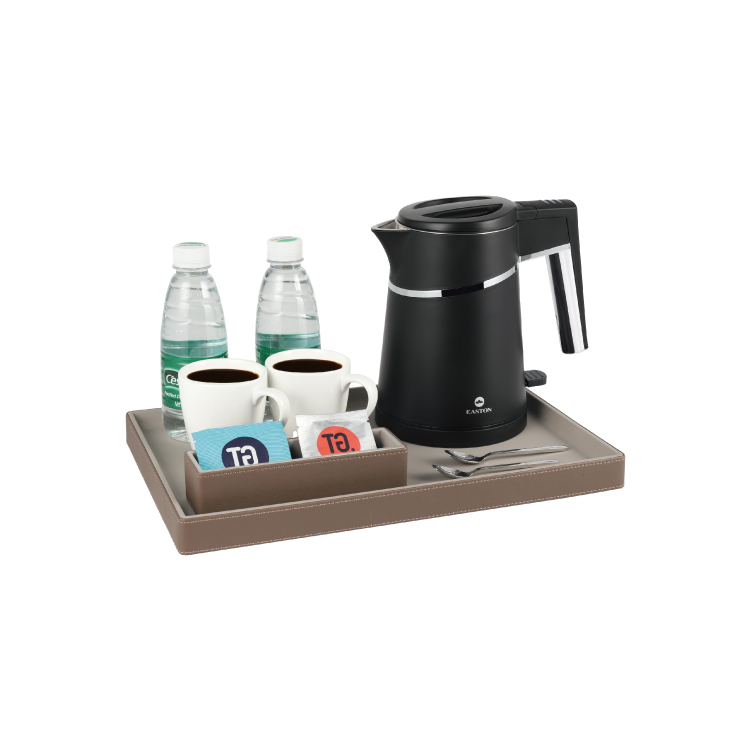The image features a detailed mock-up of a sophisticated drink tray made of light grayish-brown leather with visible white stitching. Positioned on the tray are two ceramic white coffee cups filled with dark brown coffee, accompanied by silver spoons for stirring. Alongside the coffee cups, there are two water bottles filled with clear liquid, each adorned with a green label and white cap. To the right of the bottles stands a sleek, black insulated coffee pitcher, equipped with a handle and a turn-top for easy pouring, and displaying subtle white markings and a small black button. The tray also includes a small leather container holding packets of sugar and cream in blue and white wrappers.